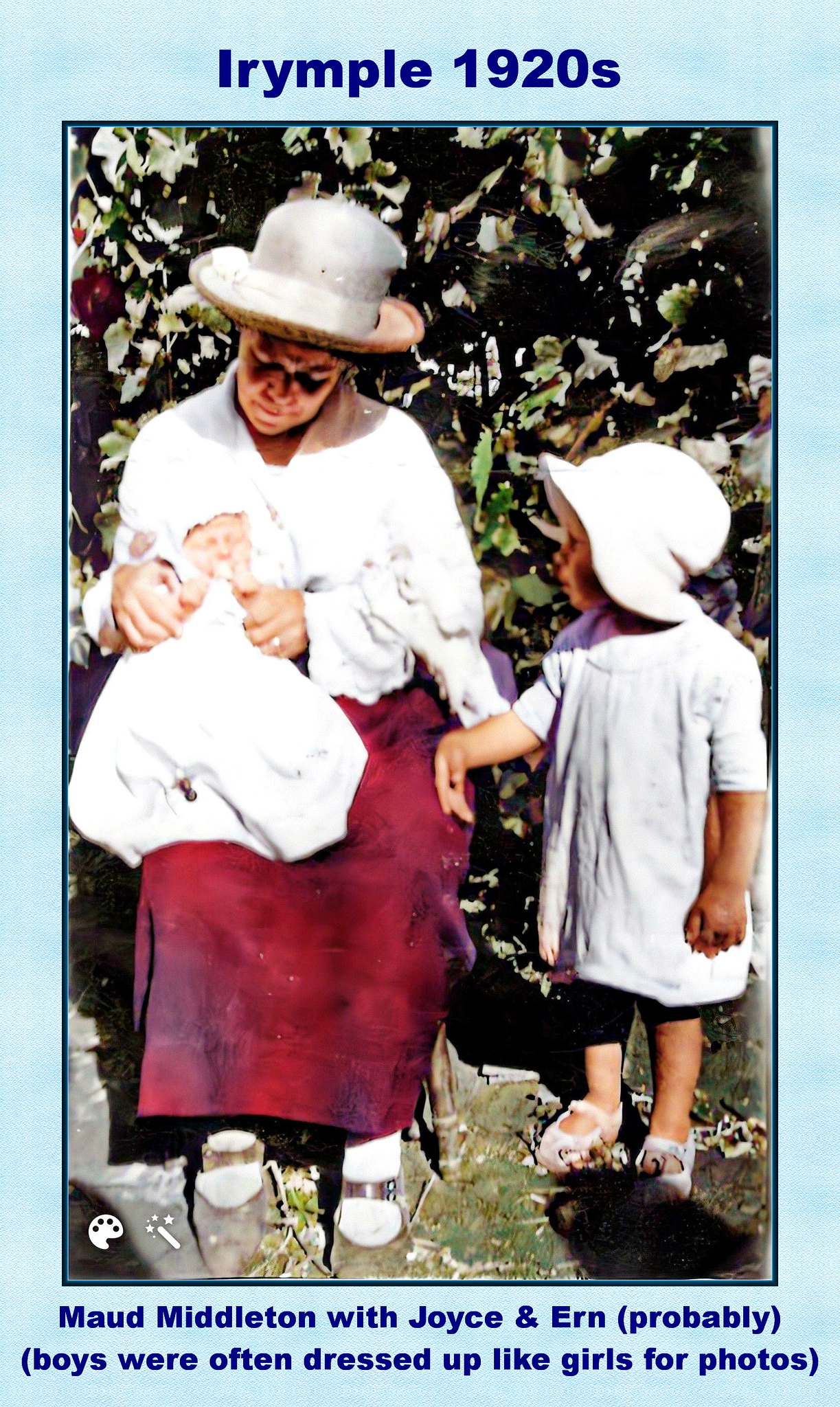An old photograph, set against a light powder blue background, captures Maude Middleton with an infant and a toddler, titled "Irimple 1920s" in dark blue lettering at the top. Below, the caption reads, "Maude Middleton with Joyce and Erin, probably boys, were often dressed up like girls for photos."

In the photo, Maude sits outdoors amidst green foliage and grass, wearing a silver hat resembling a cowboy style, a white blouse, a red full-length skirt, white socks, and Mary Jane shoes. She cradles an infant in a long white dress and bonnet, who faces the camera. Beside her stands a toddler in a short pale blue or white dress, white Mary Jane shoes, and a white hat. The scene is bathed in sunlight, highlighting their period attire and the serene outdoor setting.